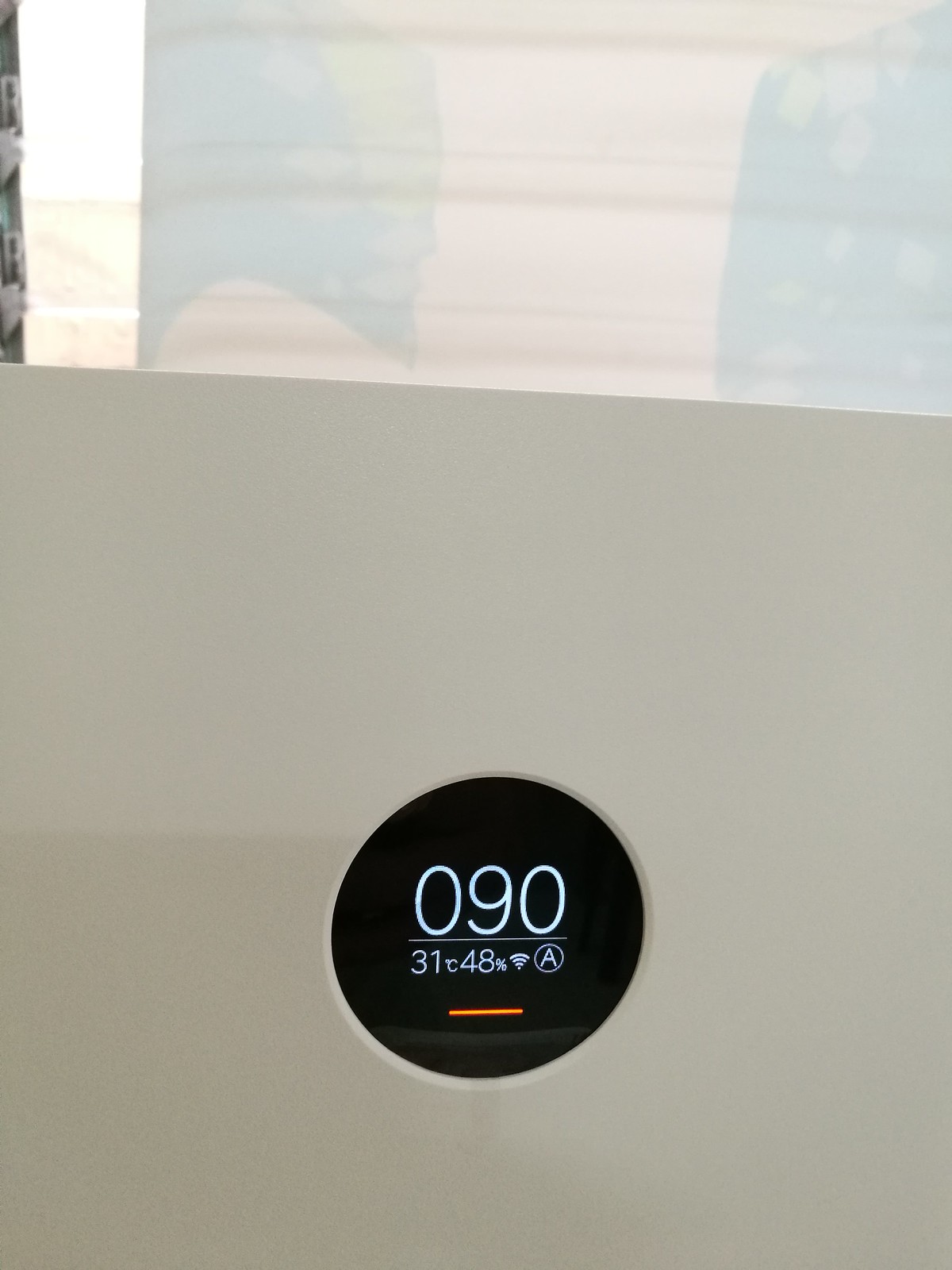The image shows a smart thermostat device, likely from a brand resembling "Airstat" or something similar. The thermostat is a white rectangular box with a circular display screen featuring black and white digital readouts. The screen displays several key indicators: "090," "31°C," "48%," along with a Wi-Fi symbol and an "A" enclosed in a circle. Below these indicators, a horizontal orange line is visible. This suggests the thermostat is actively connected to a network and possibly in an automated setting mode. Notably, the temperature is in Celsius, indicating the location is likely outside the United States.

The white box has a subtle indent on its left side, though its precise function or measurement capability remains unclear. Above the thermostat, there is a faint shadow of what appears to be a wet cloth or fabric, adding to the sense that this scene might be set in a bathroom. To the right of the shadow, there are two indistinct blue shapes accompanied by three ribbed lines, which might be part of a shower curtain or similar bathroom accessory. On the left side of the image, two white objects are hanging on the wall, though their exact nature is indeterminate.